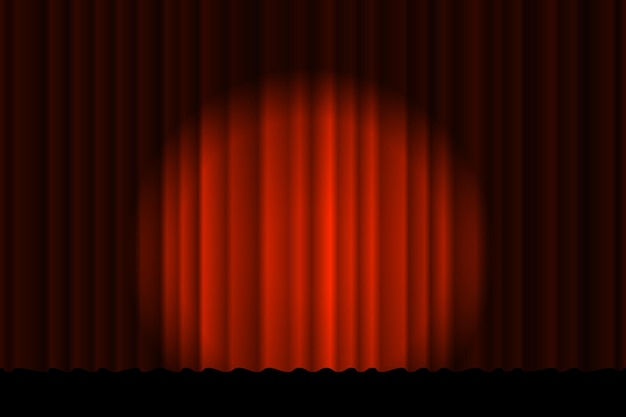The image depicts a digitally created scene mimicking a theater stage. Dominating the center is a crimson curtain, richly textured with ripples and waves, cascading down to an unseen platform. A focused spotlight dramatically lights the center of the curtain, accentuating the vibrant red hue against the darker, shadowed folds that surround it. Below the curtain, the bottom of the image is shrouded in complete blackness, offering no insight into the stage floor. The picture's predominantly red and black color palette enhances the theatrical ambiance, while no performers or text are visible, emphasizing the emptiness and anticipation before a performance.